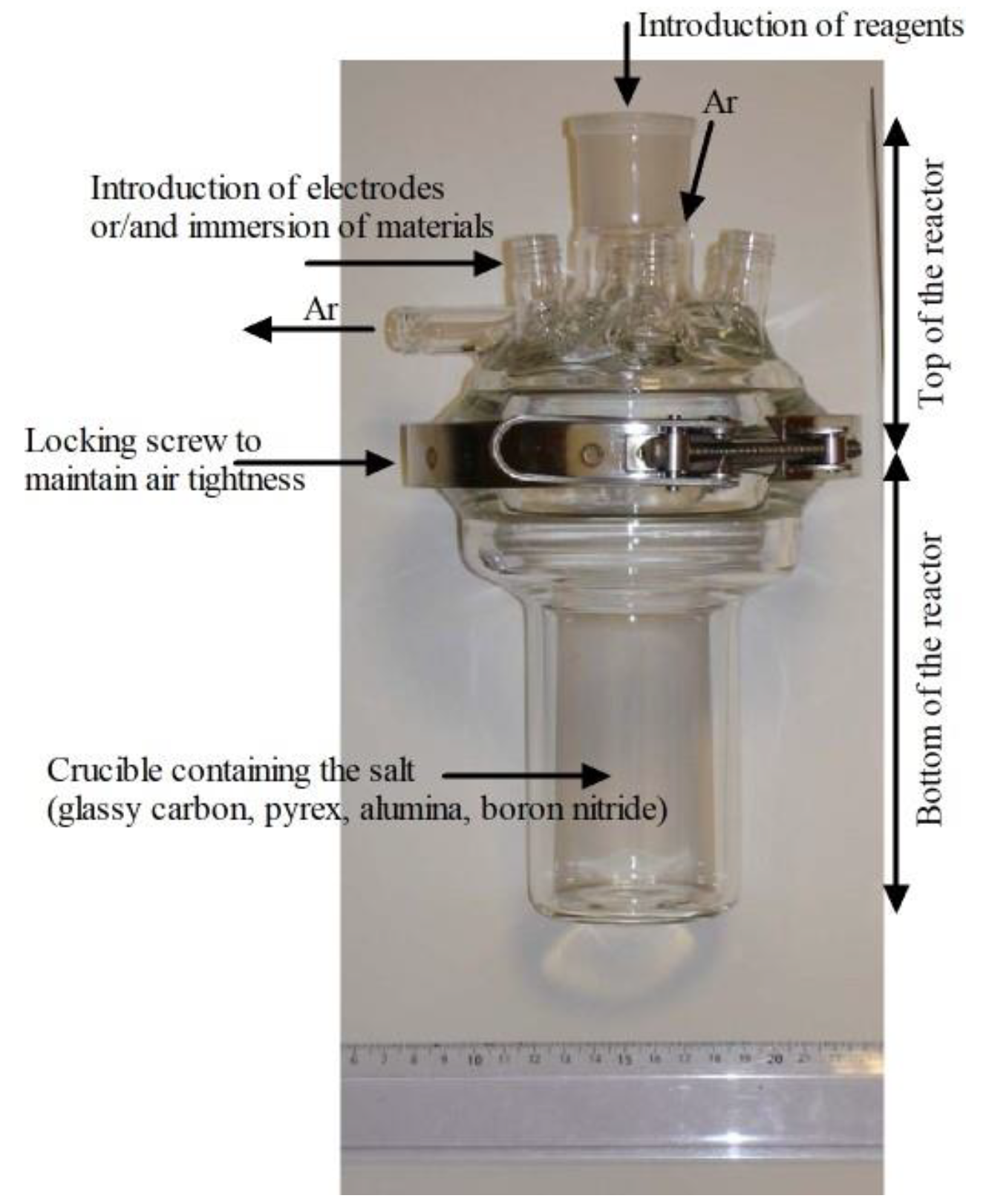This image depicts a detailed diagram of a small glass reactor used in scientific experiments, likely in a history or science class. The reactor features a tubular, transparent design with multiple layers, providing a double barrier of protection. It is equipped with a ruler at the bottom to indicate its size, though the exact measurements are not clear. The reactor comprises several distinct parts labeled with text annotations.

The base of the reactor is labeled "crucible containing the salt," specifying materials like glassy carbon, Pyrex, alumina, and boron nitrate. Above the base, the central section includes a "locking screw to maintain air tightness," which appears to be a metal component designed to secure the structure. The top section has multiple tubes for different inputs and outputs. Tubes labeled "introduction of electrodes and/or immersion of materials" and one marked "AR" project from the top and side. An arrow points to an open tube at the top, labeled "introduction of reagents." The image also has markers along the side, measuring the "top of the reactor" and "bottom of the reactor."

This detailed setup indicates that the piece of equipment is intended for creating and studying small chemical reactions within a controlled environment.